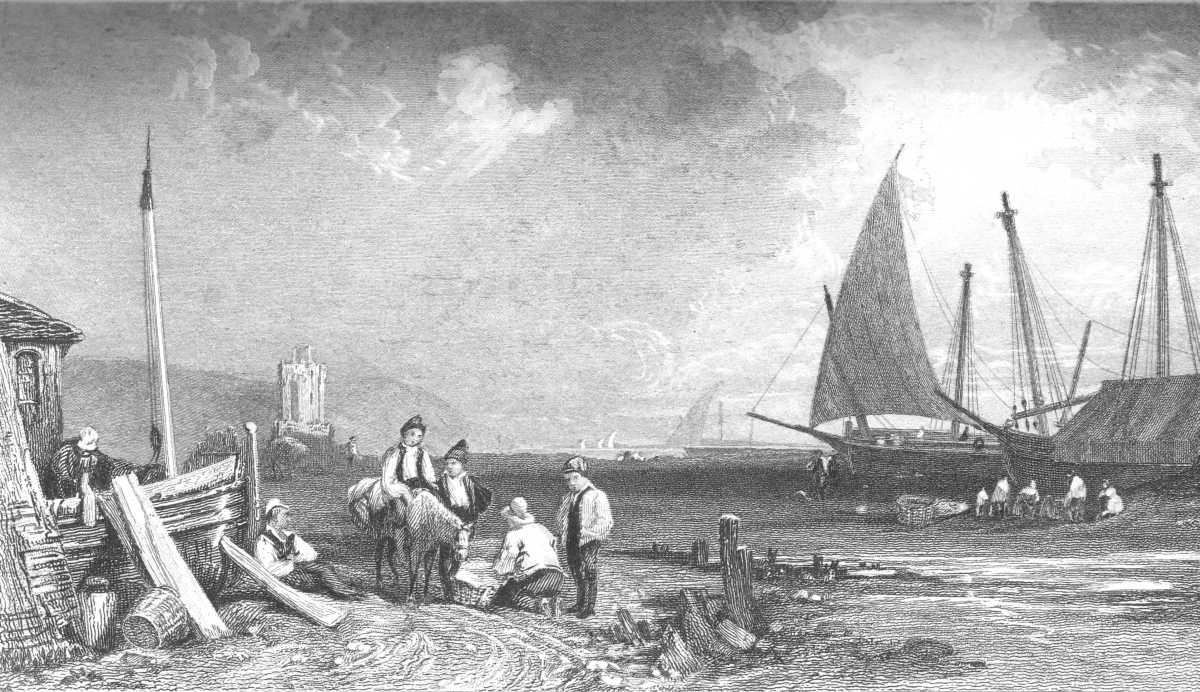This is a monochromatic, historical-looking image, likely a detailed pencil or charcoal sketch, depicting a bustling harbor scene. The sky above is filled with dark gray clouds with the sun breaking through, casting a white glow onto the land and the ocean. In the background, multiple boats sail on the water, including one large sailboat with prominent sails and masts. Closer to shore, smaller boats float in the shallow water.

On the beach and shoreline, many men in white shirts, some with hats, are gathered. They're engaged in various activities around a wooden shack or old boat, possibly repairing it. There are baskets on the shore, hinting at a mix of rescue and daily work. A man on horseback stands out among the figures, adding to the sense of activity and urgency. The shoreline scene suggests these men might have been rescued from a shipwreck.

In the distance, additional buildings and hints of mountains can be seen, alongside what appears to be a lighthouse. This intricate image captures the essence of a historical harbor, teeming with activity, set against a dramatic sky.